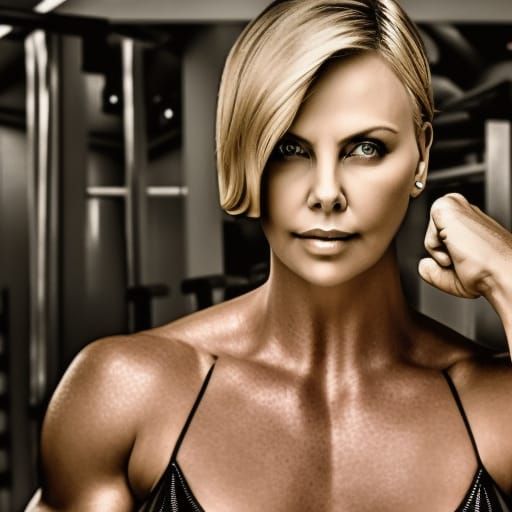The image in question appears to be a square photo that portrays a digitally altered or photoshopped depiction of Charlize Theron. The top half of the picture prominently features Theron's face with her platinum blonde, short haircut, and a faint earring on her right ear. Her facial complexion is a slightly pale, almost yellow-bronze, and she dons shiny lipstick, which gives her a somewhat artificial look. This face is juxtaposed onto the body of a highly muscular individual, one typically associated with bodybuilders, dressed in a black spaghetti strap top that seems to dissolve mid-way up the torso, suggesting digital manipulation. 

The skin tone disparity is notable, as the body below is a shiny bronze while Theron's face is paler. Furthermore, the lighting and shadows on the face and body do not align, enhancing the oddness of the composition. Her posture suggests a pose often seen in fitness photography, with her right arm lifted and clenched into a fist beside her ear, as if showing muscle. The background behind her is somewhat blurred but hints at gym equipment and grey walls, contributing to the photo's overall sense of being set in a fitness environment. Despite Theron's recognizable face, the mismatch in body and shading highlights the surreal and edited nature of the image.